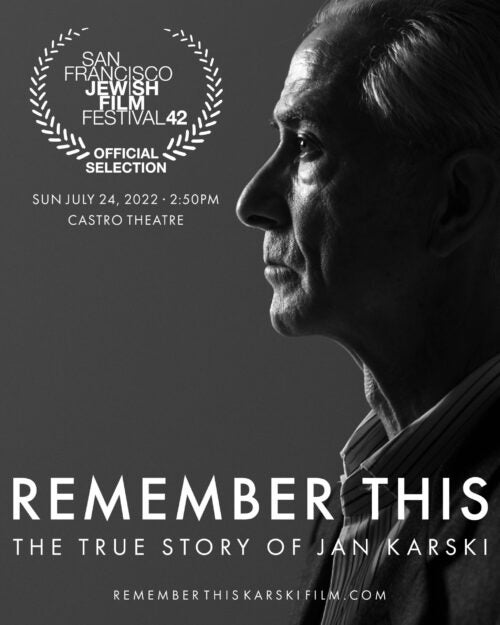The movie poster, presented in striking black and white, features a somber side profile of an older gentleman, likely in his 70s or 80s, facing left. Positioned on the right side of the poster, his pensive expression aligns with the serious tone of the image. At the top left, a logo for the San Francisco Jewish Film Festival 42 is prominently displayed, adorned with a decorative wreath on both sides. Below this, the text reads "Official Selection," followed by the event details: "Sunday, July 24, 2022, 2:50 p.m. at the Castro Theater" in small white letters. Dominating the bottom portion of the poster, the film's title "Remember This" stands out in large white text, with a subtitle beneath it in thin white letters, "The True Story of Jan Karski." At the very bottom, the website "RememberThisKarskiFilm.com" is provided, ensuring viewers can find more information about this evocative film that delves into Jan Karski's experiences, likely highlighting significant historical context, possibly related to World War II.